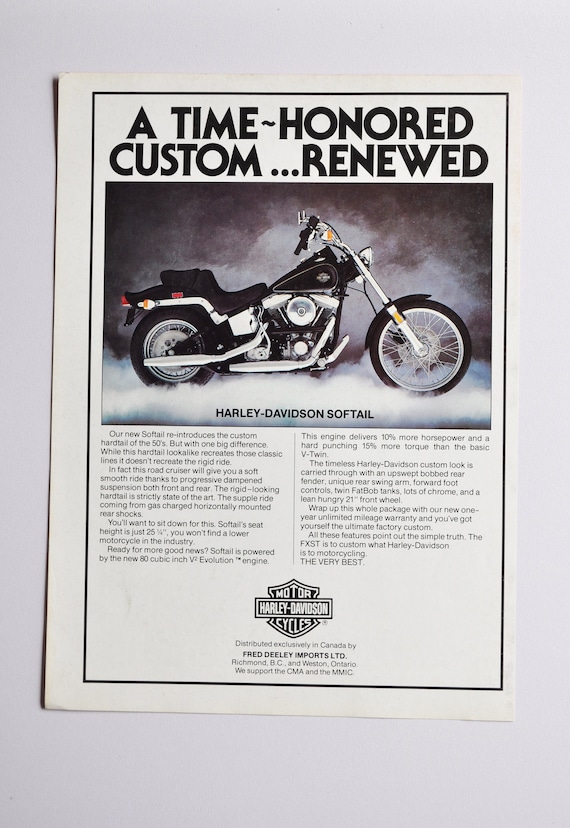The image features a prominent Harley-Davidson advertisement placed against a simple gray background. It appears as if a page has been torn from a magazine and affixed onto this backdrop. The top of the page sports a bold headline in uppercase black text: "A TIME-HONORED CUSTOM... RENEWED," encapsulated by a thin black border. 

Central to the image is a striking black and silver Harley-Davidson Softail motorcycle, with the front wheel pointing to the right and the back wheel oriented to the left. This visually rich Harley-Davidson bike, sporting a black seat and intricate silver detailing, serves as the focal point below the headline. Beneath the motorcycle image, the text elaborates on the vehicle's design, highlighting the Softail's smooth ride facilitated by its gas-charged, progressive dampened suspension, a modern take on the classic hardtail look of the 1950s.

The lower part of the ad features two columns of detailed text, divided by a thin gray line. At the page's bottom, the iconic Harley-Davidson logo — "MOTOR HARLEY-DAVIDSON CYCLES" — is prominently displayed, flanked by additional promotional content. The ad emphasizes the blend of nostalgic design and contemporary engineering that characterizes the new Softail model.